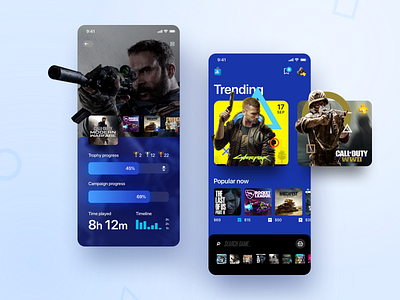The image appears to be an advertisement for Call of Duty featuring elements reminiscent of phone screens or possibly handheld game systems. On the left side, there is a long rectangular shape, potentially a phone or a game system, displaying a dark image of a man holding a gun, with the gun extending beyond the screen. At the bottom of this section, it reads "8H12M," indicating a duration, with smaller unreadable text above it. The center section shows another similar screen displaying the word "Trending," with an image of a man holding a gun, and labeled below with "Popular Now" featuring additional game icons. The right section prominently displays a square with the Call of Duty logo and an image of a helmeted soldier in an army outfit, aiming and firing a weapon. The overall color scheme has dark, blue, and brownish hues, giving a militaristic and intense atmosphere. The details also suggest mentions of other games like "World War Two" and "The Last of Us," along with indications of gameplay statistics such as campaign progress and time played.